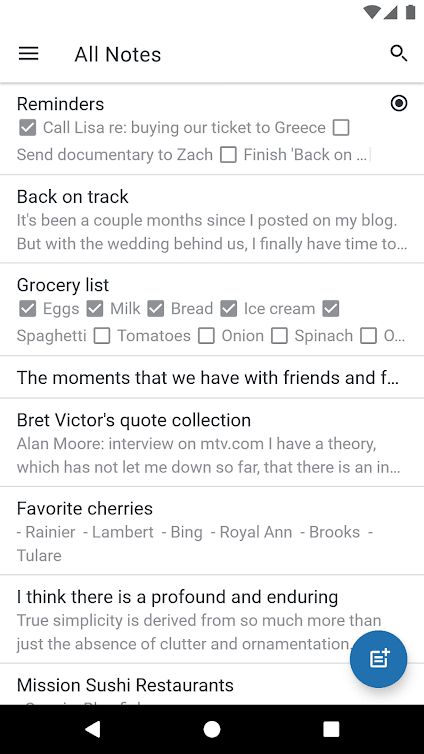Screenshot of an iPhone displaying a notes application with a predominantly white background. At the top of the screen, there are three horizontal lines indicating the menu, followed by a search icon and the text "All Notes." Below this, there are headings and entries related to reminders and tasks, some of which are checked off:

- A checked checkbox with the note "Buy no tickets to Greece."
- An unchecked checkbox with "Send document and create set."
- An unchecked checkbox with "Finish back on."

A detailed note follows, mentioning that it's been several months since the user posted on their blog but recent weather changes provided them the time to update. 

The note seamlessly transitions into a grocery list with several checked items:
- Eggs (checked)
- Milk (checked)
- Bread (checked)
- Ice cream (checked)
- Baguette (unchecked)
- Tomato (unchecked)
- Onion (unchecked)
- Spinach (unchecked)

The screen also includes a reflective narrative about life philosophies related to clutter and simplicity, mentioning "profound and enduring true simplicity" and a critique about the difficulties of being a real landlord compared to perceived favoritism.

At the bottom, there is a navigation bar with icons resembling a back arrow, a stop button, and a square. Above this bar, there is a circular icon with a musical note and a plus symbol inside it.